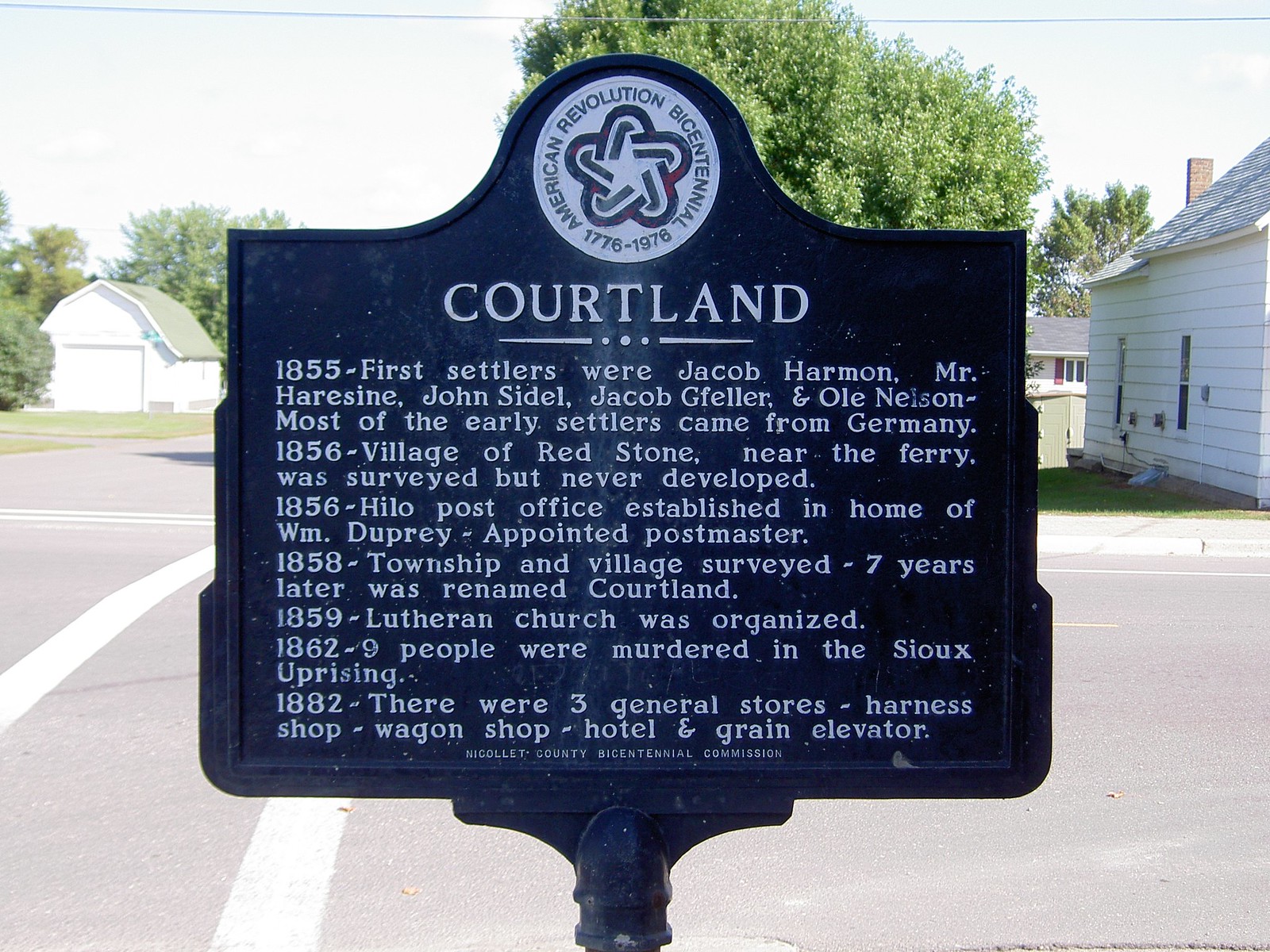This photograph captures a detailed outdoor scene centered around a prominent black metallic signboard. The signboard features a circular emblem at the top with "American Revolution Bicentennial" written around it. Below the emblem, the word "Cortland" is boldly displayed in capital white letters. Beneath this, the sign provides historical information about the area in a series of 14 lines written in white text, including notable dates and names such as "1855. First settlers were Jacob Harmon, Mr. Hairstein, John Sedell, Jacob Geffel, O. Nason" and other early historical events.

The signboard is mounted on a metal pole with a bracket that secures it in place, and there is a small holder around the bottom left, right, and underside of the sign. The pole is cut off at the bottom edge of the image.

In the background, the ground is light gray with white crosswalk lines, indicative of an intersection. Further back, there are houses, buildings, and trees lining the streets, creating a picturesque small-town setting. The sky above is a light blue, adding to the mid-day ambiance of the photograph. The overall color palette includes various shades of black, white, gray, green, orange, and red, contributing to the vibrant details of this outdoor scene.